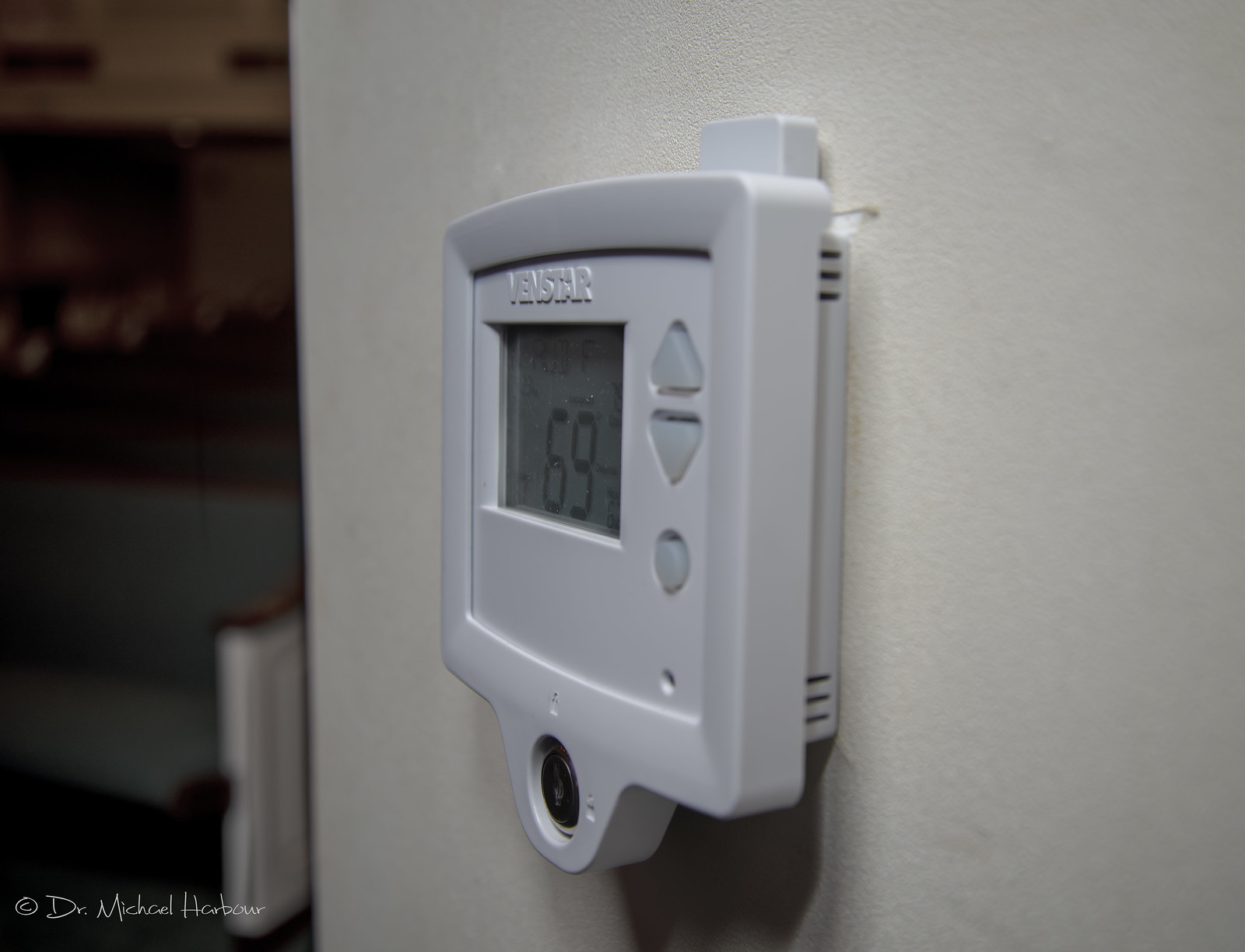Close-up of a white wall featuring a thermostat for an air conditioning unit. The thermostat, encased in a white plastic frame, is rectangular in shape. The image is taken from an angle to the right side of the device, clearly displaying the brand name "VENSTAR." The thermostat is equipped with white arrow buttons for adjusting the temperature. The digital screen shows the current temperature setting is at 69 degrees Fahrenheit.